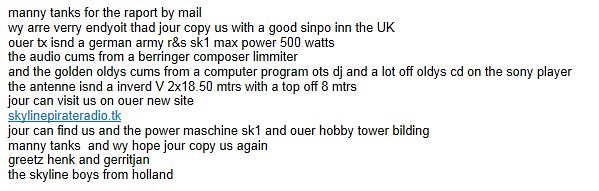The image consists of a white background with black typewriter-style text, resembling a typed-out email. The slightly flawed English hints at a translation, making it somewhat challenging to read fluently. 

The text begins with "Many thanks for the report by mail. We are very enjoy it," though the word "enjoy" appears misspelled as "ENDYOIT" in some parts. One notable feature of the text is an underlined blue link about one-third down the way, indicating a live hyperlink (skylinepirateradio.tk). 

The message continues to express gratitude for a signal report from the UK, mentioning their transmission equipment, including a German Army R&S SK1 with a maximum power of 500 watts. Audio details highlight the use of a Behringer Composer limiter and music played from a computer program (OTS DJ) and Sony CD player, focusing on golden oldies. The antenna described is an inverted V2 by 18.50 meters with a top height of 8 meters, contributing to their broadcast setup.

The email-style text concludes with greetings from "the skyline boys from Holland," Hank and Jeraton, and a hopeful note that the recipient will "copy us again." The overall look and feel suggest an informal yet detailed correspondence, outlining technical aspects of their radio setup and broadcasting gratitude.